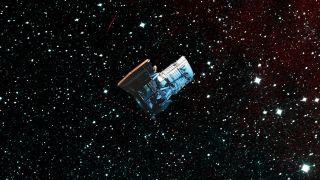The image depicts a rectangular, horizontally oriented photograph of deep space with a predominantly black background speckled with stars of varying sizes and intensities. The scene is filled with tiny, glittering points of light that evoke a sense of vast, uncharted territory. In the upper right corner, there's a distinctive red hue, suggesting proximity to a galaxy or a star cluster. Situated in the middle of this cosmic tableau is a small, white or silver object resembling a satellite. This satellite features a dark brown, reddish panel and is angled upward to the right, appearing to float serenely through the expanse of space. Among the many stars dotting the scene, a particularly larger star stands out in the bottom right corner. The overall composition gives a sense of a solitary, advanced piece of technology navigating the boundless universe, capturing the majesty and mystery of space exploration.